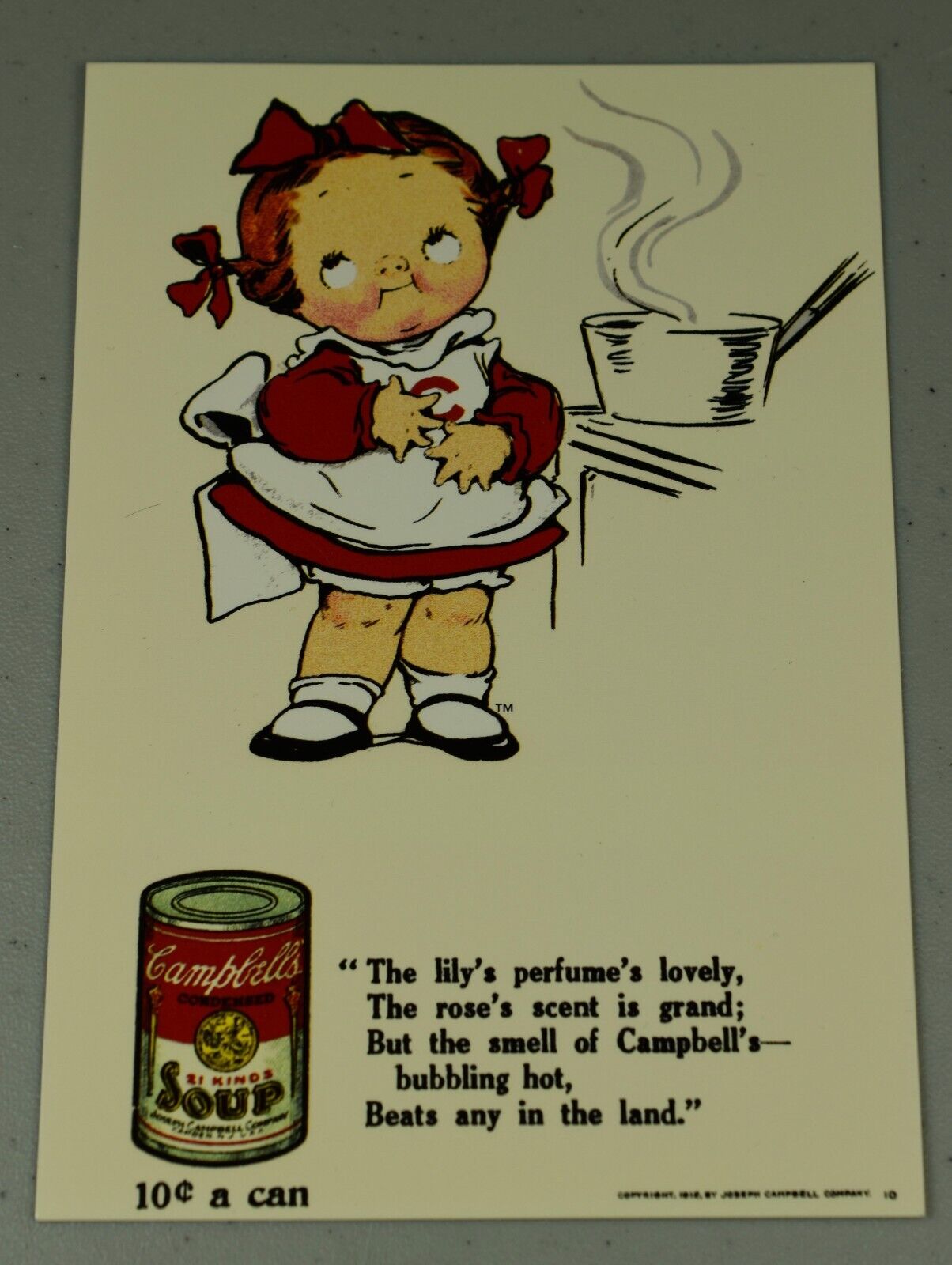This vintage Campbell's Soup advertisement, set against a dark gray background and shown in portrait orientation, depicts a nostalgic image of the iconic Campbell's Soup kid. The background of the ad is an aged yellow color. At the top left, the chubby-cheeked, pigtailed girl with red hair adorned with red bows is dressed in a red dress and a white apron emblazoned with a red "C." She is portrayed with her hands over her chest and stomach, her oval eyes looking upwards as if savoring the thought of the delicious soup. Her attire is completed with black Mary Jane shoes and white socks, one of which is turned down.

Next to her, a minimalist graphic of a stove features a small saucepan with steam rising, indicating the warmth and aroma of Campbell's soup. The advertisement's lower section includes an illustration of a Campbell's Soup can, priced at 10 cents, accompanied by a whimsical poem: "The lily’s perfume’s lovely, the rose’s scent is grand, but the smell of Campbell's bubbling hot beats any in the land." This detailed composition captures the charm and essence of vintage advertising, highlighting the delicious and comforting nature of Campbell's soup.